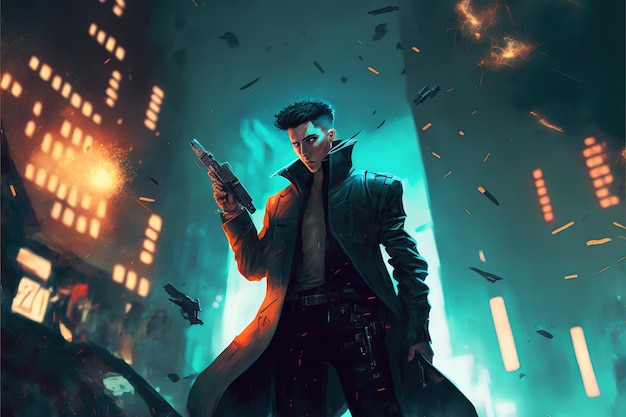In the animated video game scene, a spy-like figure is depicted in the center amidst urban chaos. The background features dark-colored buildings lined on either side, their somber facades punctuated by brightly lit windows in shades of orange and yellow, suggesting they are illuminated from within. The figure, clad in a long, dark trench coat, holds a gun in his right hand while his left hand clutches the hem of his coat, revealing an arsenal of metallic weapons strapped to his leg. He wears a belt and has short black hair, reinforcing his stealthy, enigmatic aura. To the right and left of him, explosions illuminate the night, casting an orange glow and sending debris flying through the air, adding a sense of imminent danger and tension to the scene. Shattered fragments, primarily in black with fiery undertones, swirl around, intensifying the atmosphere of destruction.